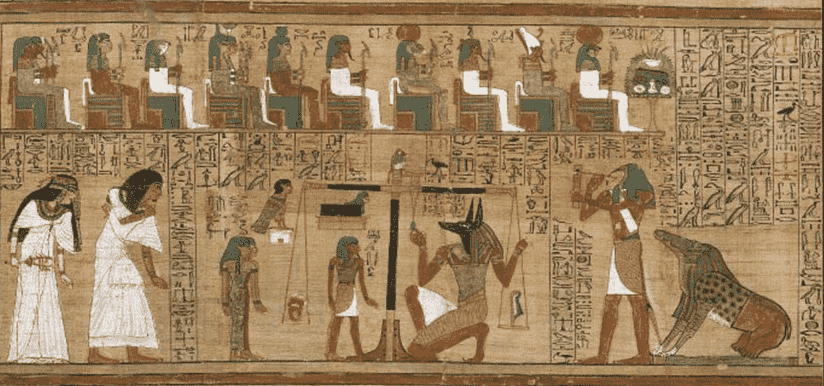In this faded but richly detailed ancient Egyptian painting, a tableau of hieroglyphs and colored drawings unfolds, predominantly in browns and whites with hints of additional colors lost to time. The top section features ten seated figures, all facing right, their attention seemingly directed towards a stack of books or scrolls. Below them, an intricate display of sacred symbols and scenes comes to life.

Central to the lower depiction is the jackal-headed Anubis, the god associated with mummification and the afterlife, standing near a large cross and a balanced set of scales, emblematic of the judgment of souls. Nearby, conspicuously active, is a stork-headed figure, likely Toth, the god of knowledge, engaged with what appears to be a scientific instrument, perhaps taking measurements. Close to Toth is a figure with an alligator head, suggesting the presence of Set, the god known for chaos and disorder.

Additionally, two large figures in white and two smaller dark-clad figures stand solemnly, all facing right and collectively observing the balancing scales. To the right of this vignette, another canine-headed deity faces left, alongside a humanoid form engaged in an act that may involve blowing into an object.

Overall, the painting meticulously combines depictions of deities, mortals, and meaningful symbols, conveying a narrative steeped in Egyptian myth and theological perspective on life, judgment, and the afterlife.